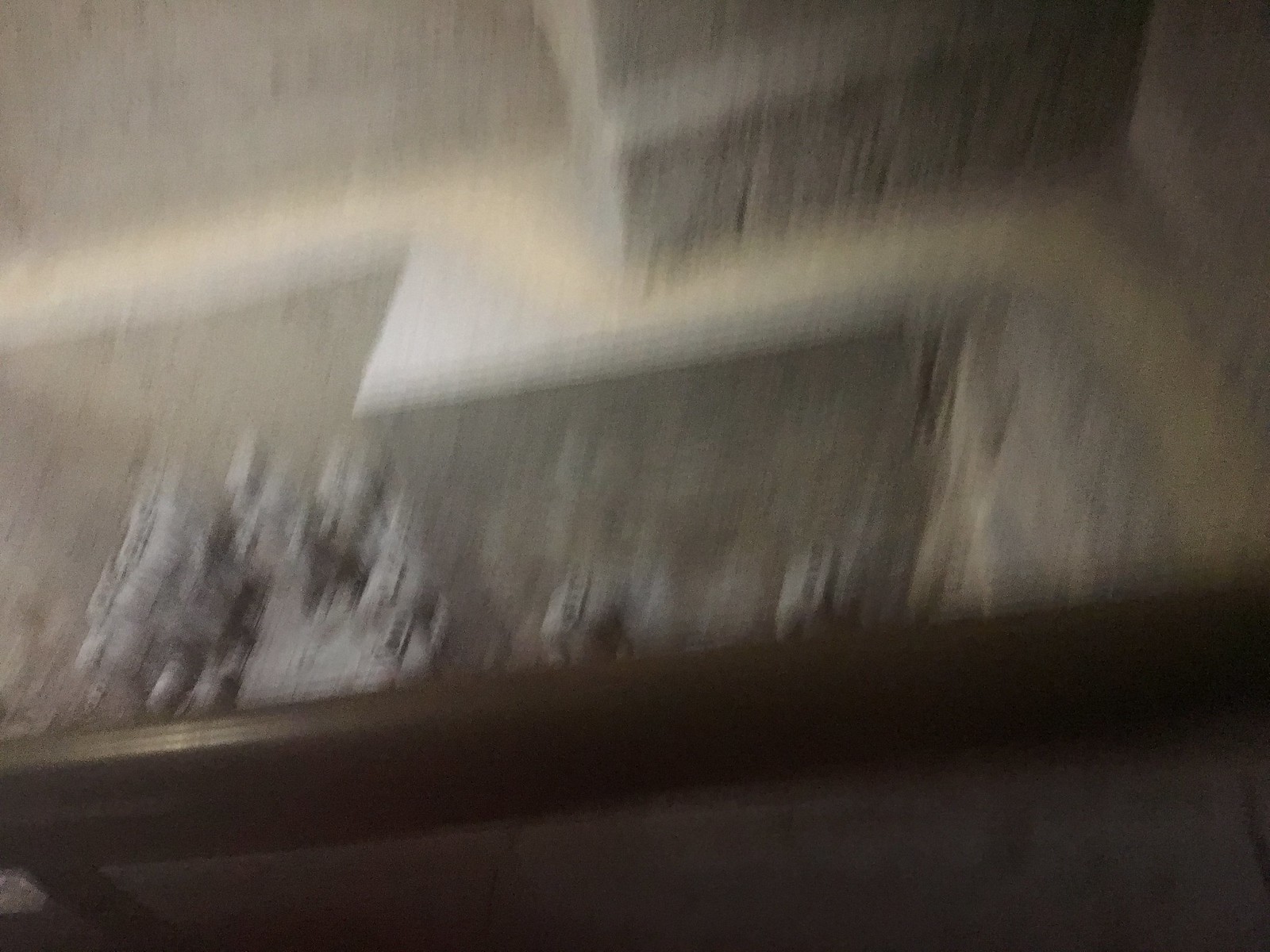This indoor photograph, taken with a blurred and streaky effect, captures an upward perspective toward a ceiling. A dark brown wooden shelf extends diagonally from the lower left corner across to the near-mid right side. Atop the shelf rest gray, rock-like, pointy structures, which are distinctly larger on the left side than on the right. These formations are unique and solitary in appearance. Along the ceiling, white crown molding adds an elegant border. Additionally, near the upper center of the image, a mysterious white angular object protrudes, contrasting sharply against the ceiling’s surface.